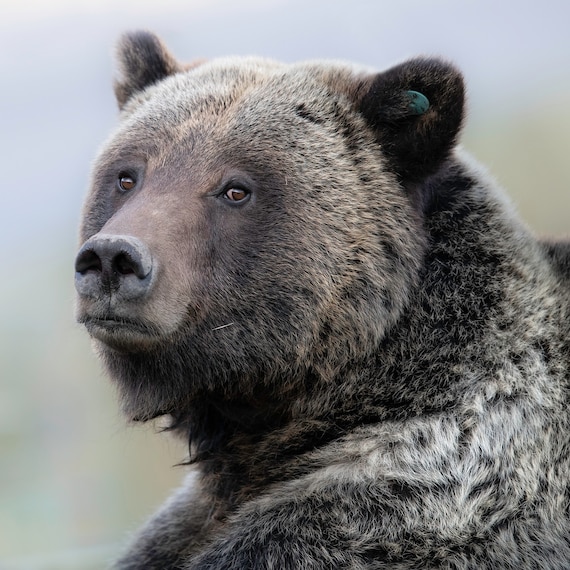This close-up image captures a brown bear with fur in varying shades of brown, dark gray, and black, accented by some white near its neck. The bear occupies about three-quarters of the frame and is presented in a diagonal side view, with its head turned towards the camera, allowing for a clear view of its facial features, including its brown eyes and nose. Its ears are a darker brown, and a subtle green tracking tag is visible inside its left ear, partially hidden by fur. The detailed focus on the bear's head and upper torso showcases its rich, multi-colored fur, suggesting preparedness for hibernation. The background is blurred, hinting at a mix of blue sky and indistinct greenery, emphasizing the bear and giving the photo a serene, natural atmosphere. Overall, the bear presents a gentle demeanor in this well-composed shot.